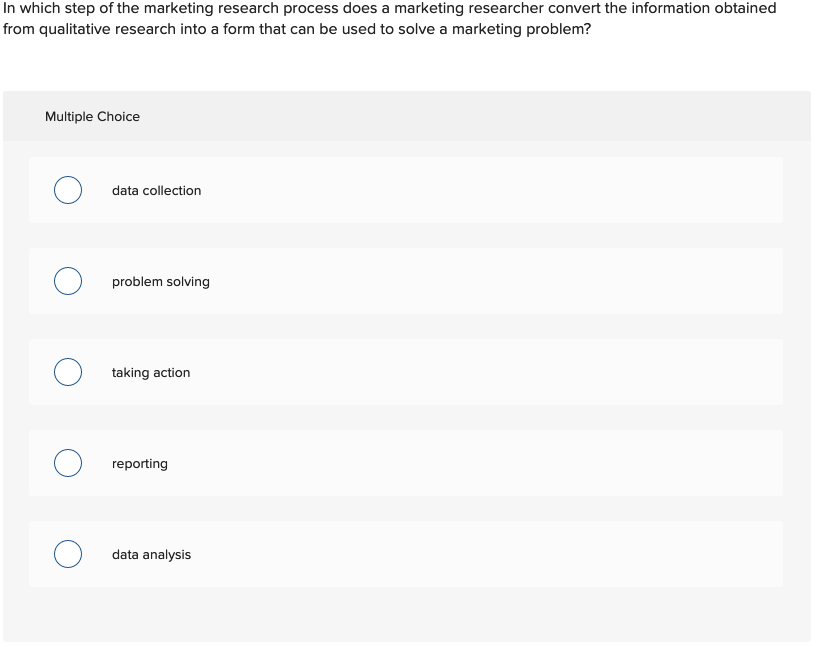This black and white image presents a step in the marketing research process, emphasizing the conversion of qualitative research information. The top of the image poses the question: "In which step of the marketing research process does a marketing researcher convert the information obtained from qualitative research into a form that can be used to solve a marketing problem?" Below this question, a large gray box labeled "Multiple Choice" houses several smaller rectangular options on the left-hand side. Each option features a white circle outlined in blue next to it, suggesting that they are selectable. The options listed are:

1. Data Collection
2. Problem Solving
3. Taking Action
4. Reporting
5. Data Analysis

The grayscale nature of the image provides no additional scenes, pictures, or colors. The source or context of this question remains unspecified beyond the "Multiple Choice" heading.